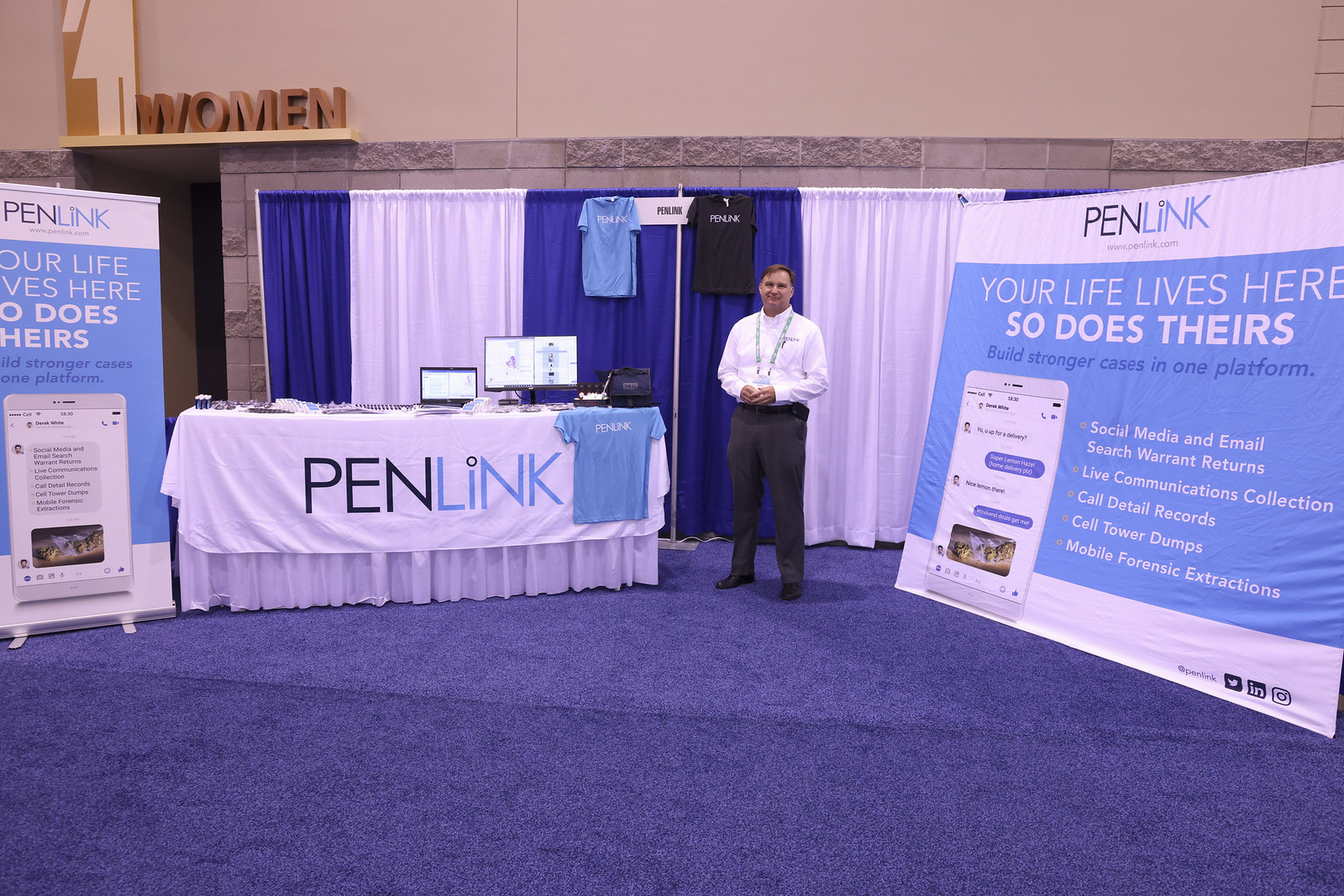The image depicts a professional networking event, likely a conference, featuring an exhibition booth for PenLink. The booth is set up in a neatly carpeted area with well-polished, blue carpeting. A man dressed in a white long-sleeve dress shirt, grey slacks, black dress shoes, and a blue lanyard stands in front of the booth with his hands folded in front of him, looking towards the camera. The booth itself is draped with a white tablecloth that prominently displays the PenLink logo, with 'Pen' in black text and 'Link' in light blue text.

In the background, there are dark blue and white curtains from which light blue and black t-shirts bearing the PenLink logo are hanging. To the left and right of the man, there are informational banners explaining the capabilities of the PenLink platform. The banners feature text such as "Your life lives here, so does theirs" and "Build stronger cases in one platform," indicating that PenLink is a tool for managing social media, email, search warrants, live communication collections, call detail records, cell tower dumps, and mobile forensic extraction. Additionally, a women's restroom sign is visible on the far left of the image, featuring a stick figure in a skirt.